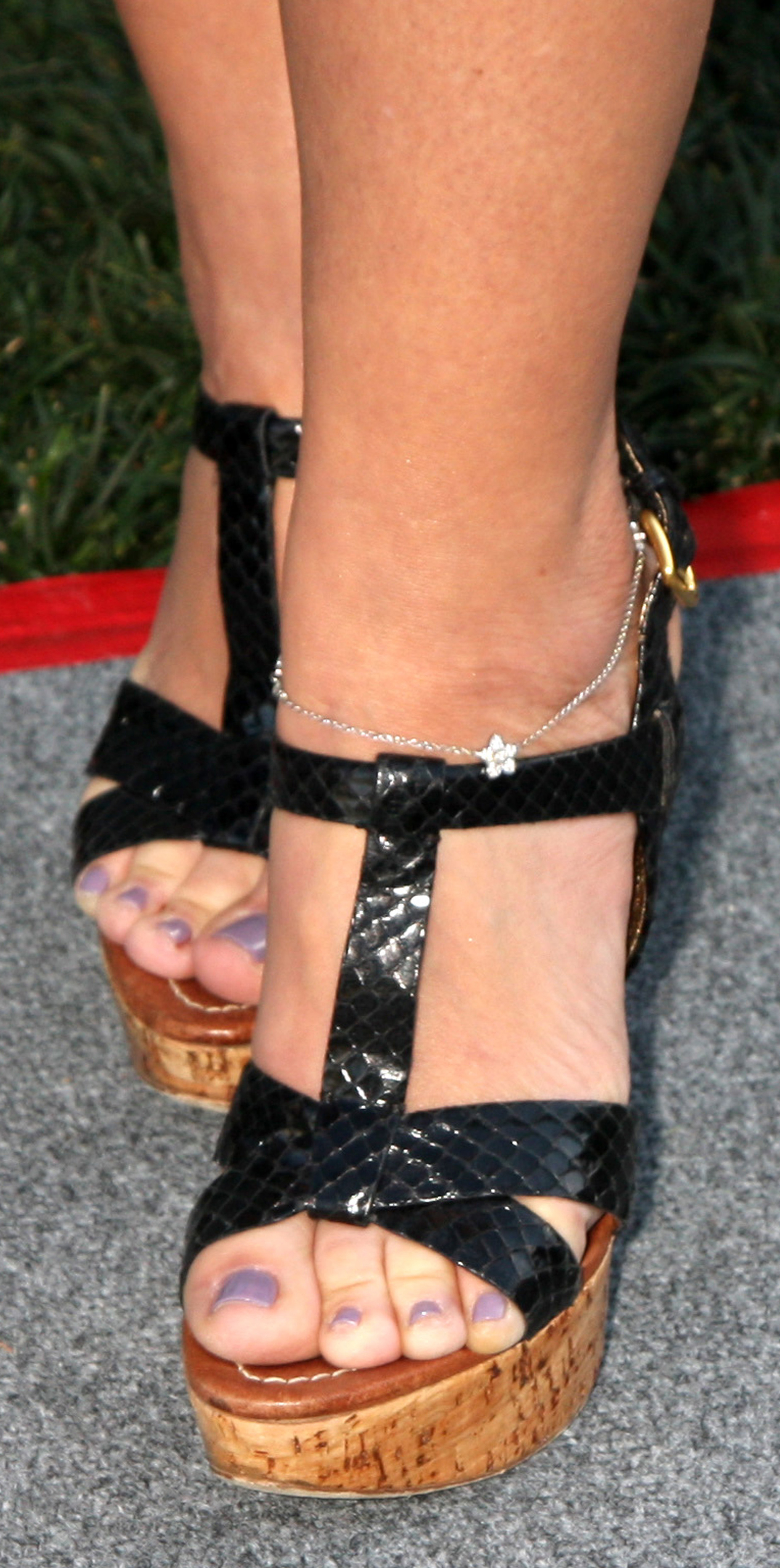The image features a close-up of a woman's ankles and feet, highlighting several details. She has fair skin and is adorned with an ankle bracelet featuring a star on her left foot, positioned on the right side of the picture. Both feet are encased in black strappy shoes with a thick, foam-like base, presenting a snake skin pattern and a gold buckle. Her toenails are painted a vivid lilac color. She stands on a mottled gray carpet, and in the background, there is a noticeable red stripe and patches of green grass.